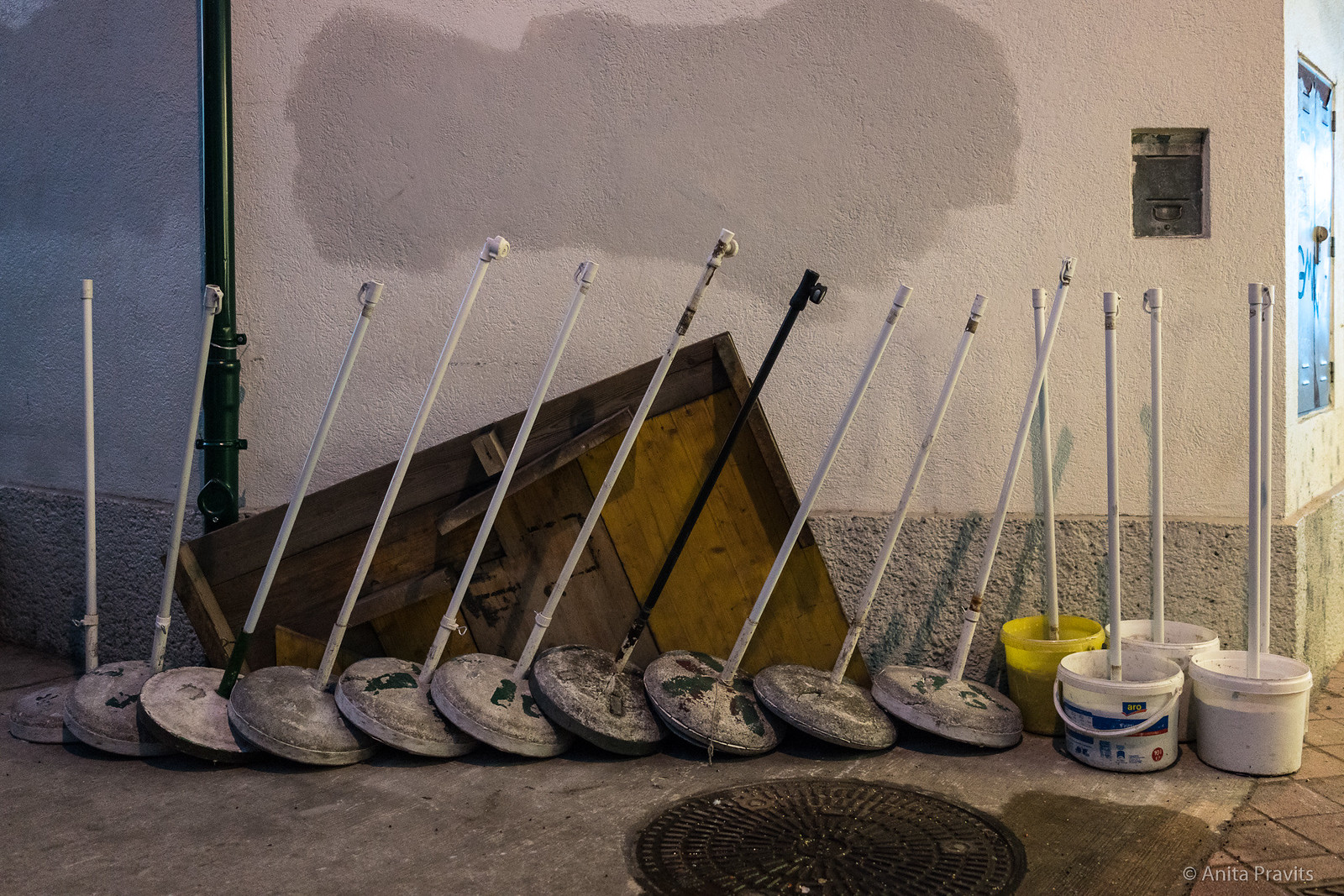The image captures a nighttime scene on a city street, featuring the side of a white building with several gray paint blotches and a pebbled textured base. Propped against the building is a large, battered wooden plank or broken door, exhibiting a patchwork of shades from white to dark. In front of this building, on the gray cement sidewalk, there are approximately 15 metallic pedestals with weathered, circular bases, each supporting long white rods capped with white. These pedestals are loosely arranged in a line, some overlapping and tilted towards the right. To the right of these pedestals, there are four buckets: three white (including one with a blue design) and one bright yellow. Each bucket also contains a white rod with a white cap. The scene also includes a circular, metallic storm drain in the foreground. Notable additional elements include a green drain pipe running down the left side of the building and a partial view of a roof and a blue object (possibly a sign or window) at the front.